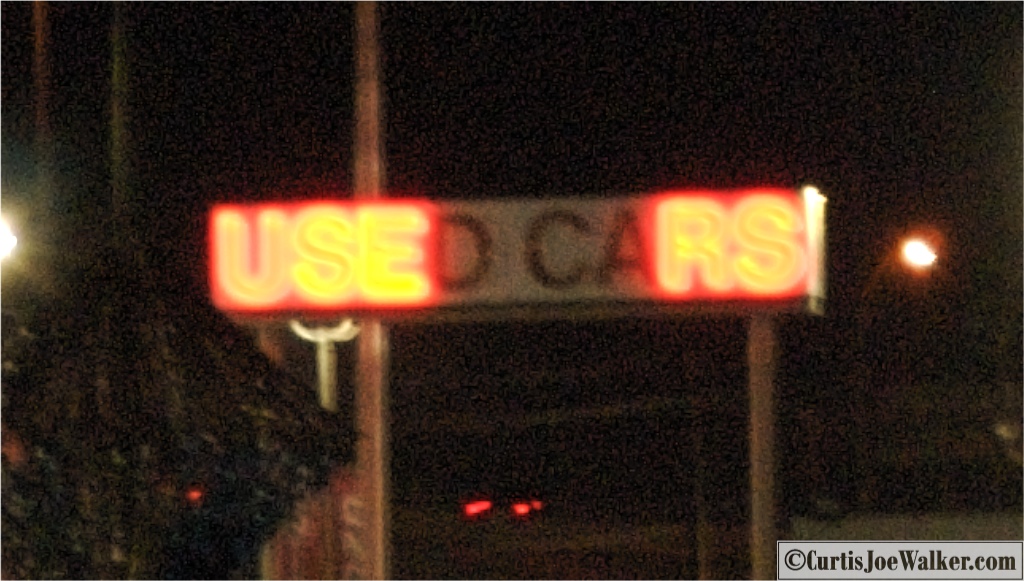A rectangular nighttime photograph prominently features a neon sign advertising "Used Cars." The image captures the long side of the rectangle from left to right. The sign, which is affixed to a set of poles, displays vibrant yellow lettering against an orange-red background. However, a noticeable section of the sign, spanning from the letter 'D' to 'CA,' is blacked out, likely due to a malfunction. The sky above is pitch black, emphasizing the time of night. In the background, additional lights can be seen on the upper right and left sides, adding subtle illumination to the scene. At the bottom right corner of the image, a watermark reads "© CurtisJoeWalker.com" in black text set against a gray background.